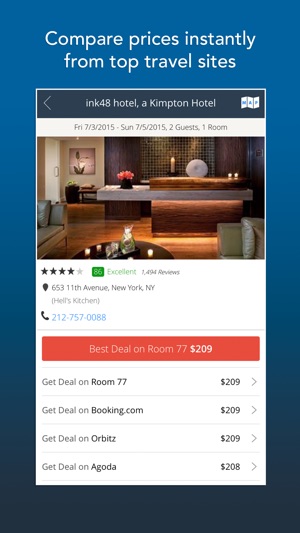**Detailed Caption:**

The mobile app screenshot features a visually appealing gradient background transitioning from a lighter blue at the top to a darker navy blue at the bottom. Prominently displayed in the top middle portion, the app invites users to "compare prices instantly from top travel sites." Just beneath this text, on a navy blue background, the app highlights "Inc. 48 Hotel, a Kimpton Hotel."

To the left of this hotel name, a left-facing arrow, likely serving as a back button, sits adjacent to a timestamp indicating a stay from Friday, July 3, 2015, to Sunday, July 5, 2015, for two guests in one room. The center of the screenshot showcases an inviting image of a serene, zen-like room adorned with numerous flowers on a wooden table. The table, which appears to have a glossy varnish, suggests it might be made of dark wood, possibly mahogany or dark maple. Nearby, candles add to the tranquil ambiance, and the presence of a wooden bathtub enhances the overall zen quality.

A comfortable sofa set is positioned to the left of the wooden table, accompanying a circular table topped with additional candles. Below this tranquil scene, the hotel boasts a rating of four black stars out of five, with an impressive score of 86 for 'excellent' based on 1,494 reviews. The hotel's address is clearly listed as "653 11th Avenue, New York, New York, Hell's Kitchen," along with a contact number: 212-757-0088.

At the bottom of the screenshot, a highlighted rectangle emphasizes that the best deal available for Room 77 is priced at $209.